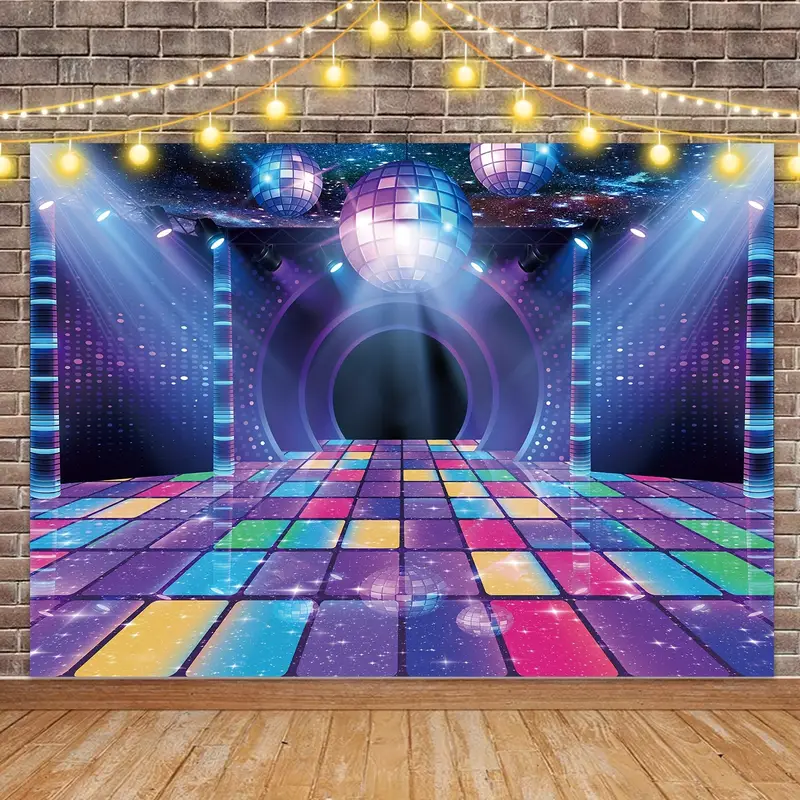This is a color photo of a large, life-size 3D mural poster hanging on a light purplish-toned brick wall. The dynamic and vibrant mural depicts a colorful disco scene with three reflective disco balls hanging at the top, casting rays of light onto the multicolored dance floor below. The floor is composed of a grid-like pattern of squares in various colors including purples, blues, yellows, pinks, and greens. Spotlights and strobe lights shine down onto the floor, enhancing the lively atmosphere. An optical illusion in the center of the mural creates the appearance of a rounded arch that seems to go deeper into the wall. In front of the mural is a light wooden floor. Twinkle lights, including larger round ones in the foreground and smaller ones in the background, hang from the top and frame each side of the mural poster.